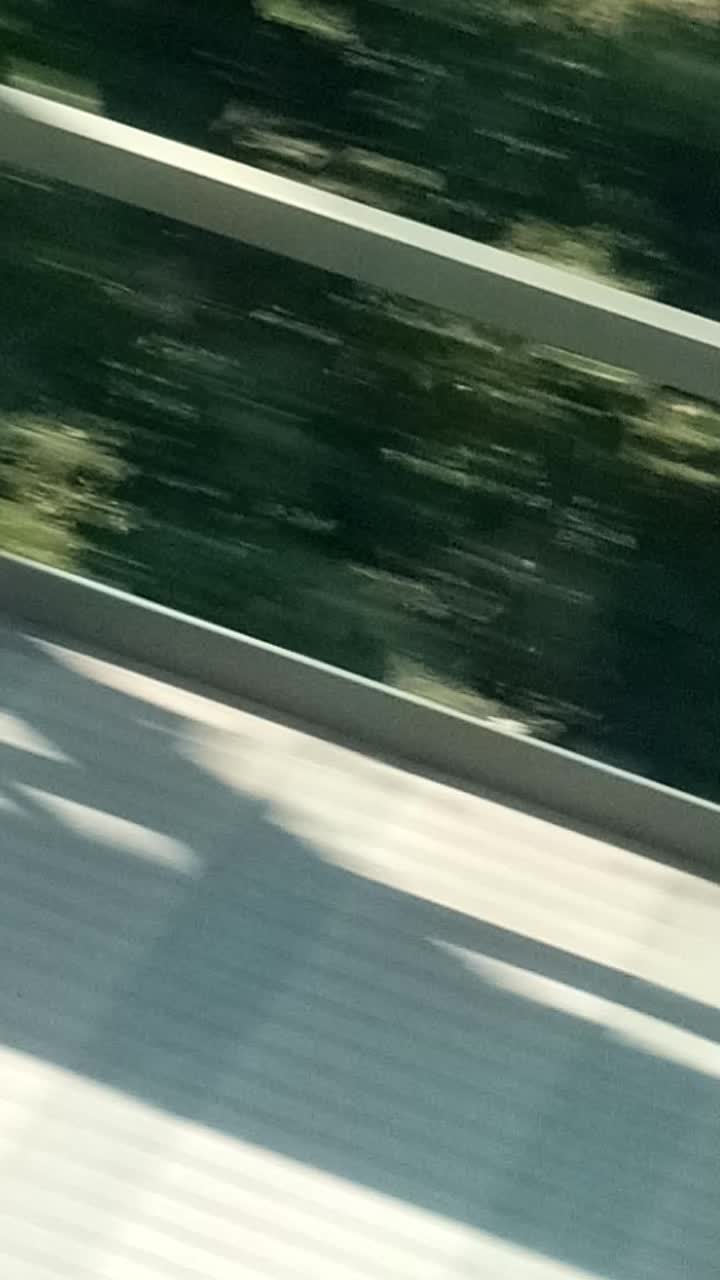The image appears to be a quickly taken, blurry photograph resembling a "drive-by" shot. The foreground features the bottom portion of a structure that looks like a white metal bridge. The details are unclear, but the bridge's material gives off a metallic sheen. In the background, on the right side, there's a collection of greenery comprising various shades of green, including dark, light, and a hint of yellow-green, indicating a mix of trees or foliage. Additionally, there's a white bar—possibly wooden—visible within the scene. A shadow is discernible at the very bottom of the bridge, though its source is ambiguous due to the rushed nature of the photo.